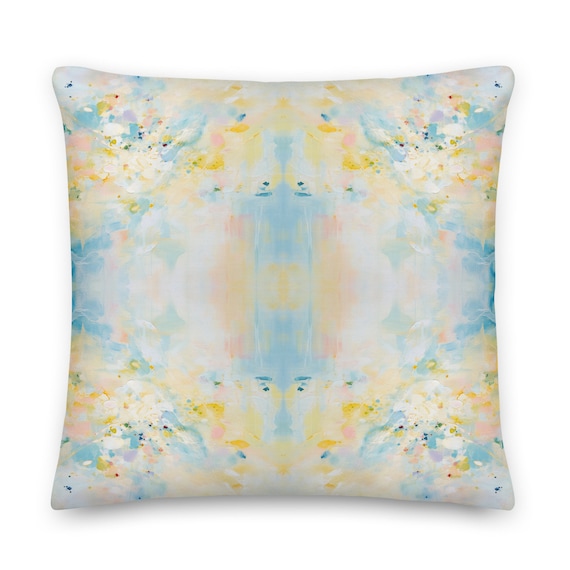In this image, we see a distinctive square pillow with slightly irregular edges, giving it an artistic, handmade appearance. The background is light gray, featuring a vibrant, abstract watercolor design. The predominant colors are bright blue, light orange, and yellow, with subtle touches of pink, purple, and white. The pattern appears more concentrated in the center, where there is an interplay of blue and orange hues creating a slightly blurred effect reminiscent of blotting. Towards the edges, the colors appear sharper and more defined, with darker flecks of blue particularly noticeable in the corners. The central section also seems to have a vertical and horizontal blur, forming a cross-like shape. This design, with its varied, colorful flecks and soft blurs, gives the impression of a carefully crafted, painted pillow.